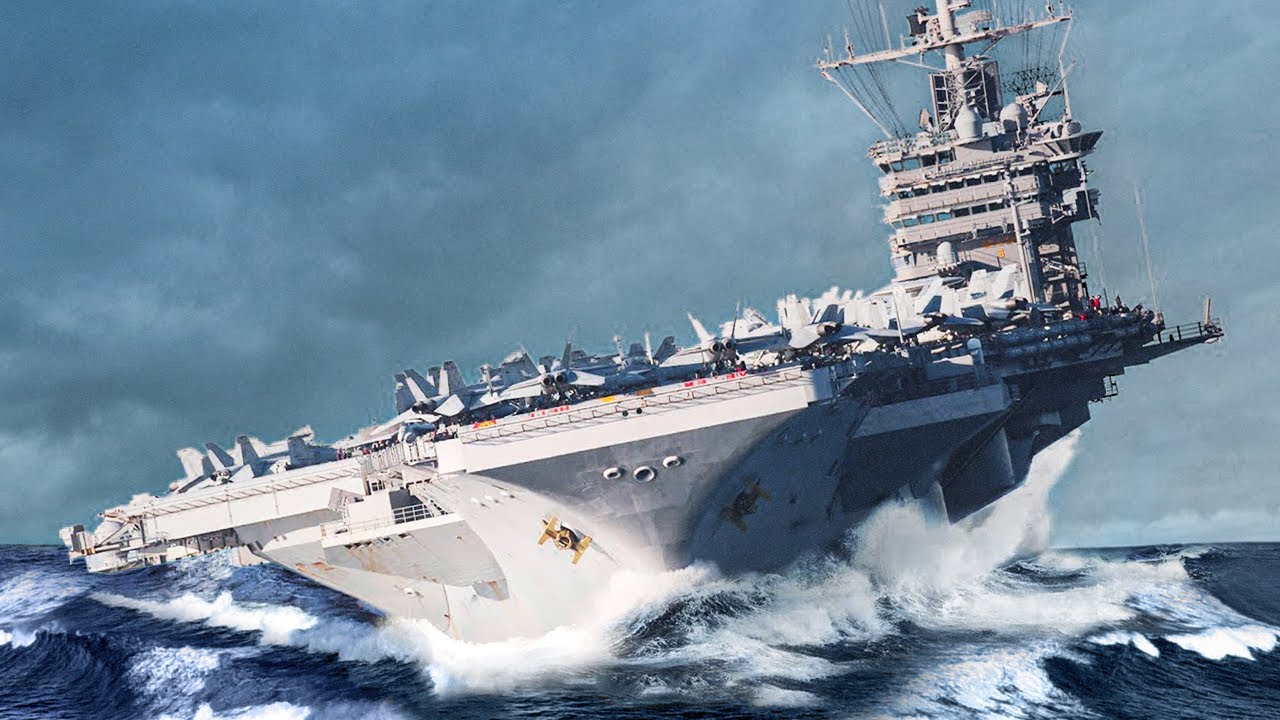This image, possibly an extremely detailed painting or a photograph, portrays a dramatic maritime scene under a blue and gray sky. The ocean below features dark blue, turbulent waters with white-capped waves and foam. Central to the composition is an enormous aircraft carrier, tilted such that its left side is closer to the water. The ship, primarily white and gray with a flat top surface, resembles a floating naval base, loaded with numerous light gray and almost white fighter jets securely parked towards the front. The carrier's distinct structure includes a towering communication tower at the back right, featuring multiple levels, rows of windows, and an array of wires and antenna-like structures. The background reveals a darker blue sky in the upper left corner, blending with lighter clouds, enhancing the overall maritime environment's intensity.